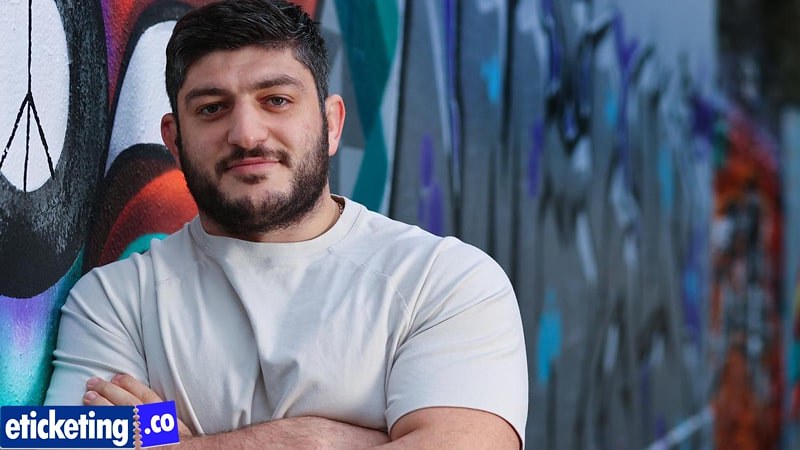The image portrays a muscular man with tanned skin, brown hair, a black beard with hints of gray, and a moustache, leaning against a meticulously painted graffiti wall. He is dressed in a white short-sleeved T-shirt and stands with his arms folded across his chest, showcasing a subtle, straight-across smile. The graffiti backdrop is organized and appears to be a deliberate mural, featuring a well-defined peace symbol with a thick black border on the left side, alongside various other colorful elements, including a snake-like image with orange, black, and white bands, and traditional graffiti taggings that blur into the background. In the lower left corner of the image, there is a blue banner designed to resemble a ripped ticket, with "e-ticketing" written in white text on the dark blue part and ".co" on the lighter blue part.